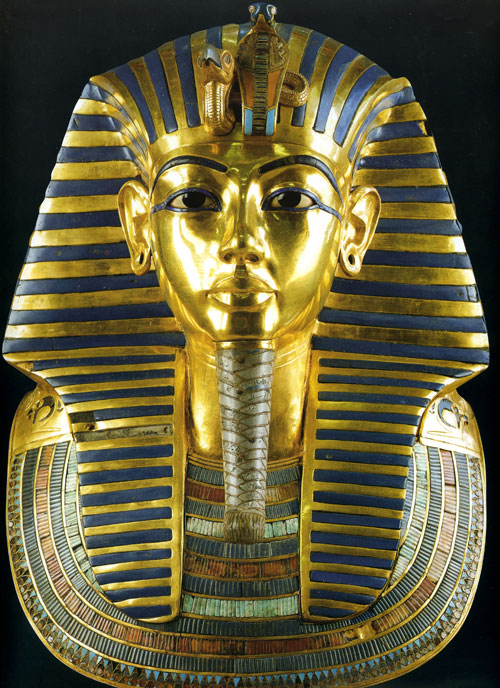This detailed image captures a golden statue of an Egyptian pharaoh, possibly representing King Tutankhamun. Set against a stark black background, the statue’s headdress is adorned with mesmerizing blue and gold stripes that run horizontally across the sides and vertically over the top and back. The face of the statue, framed by the striped headdress, features strikingly dark black eyebrows arched above blue-lined eyes. The pharaoh's earlobes are decorated with earrings. Hanging from the chin is a grayish braided structure that may symbolize a ceremonial beard. The neckpiece of the statue is elaborately designed with striations and mosaic-like inlays of blue, green, orange, and red stones, giving it a vibrant and intricate appearance. This close-up shot emphasizes the exquisiteness and opulence of the artifact, highlighting its historical and artistic significance.